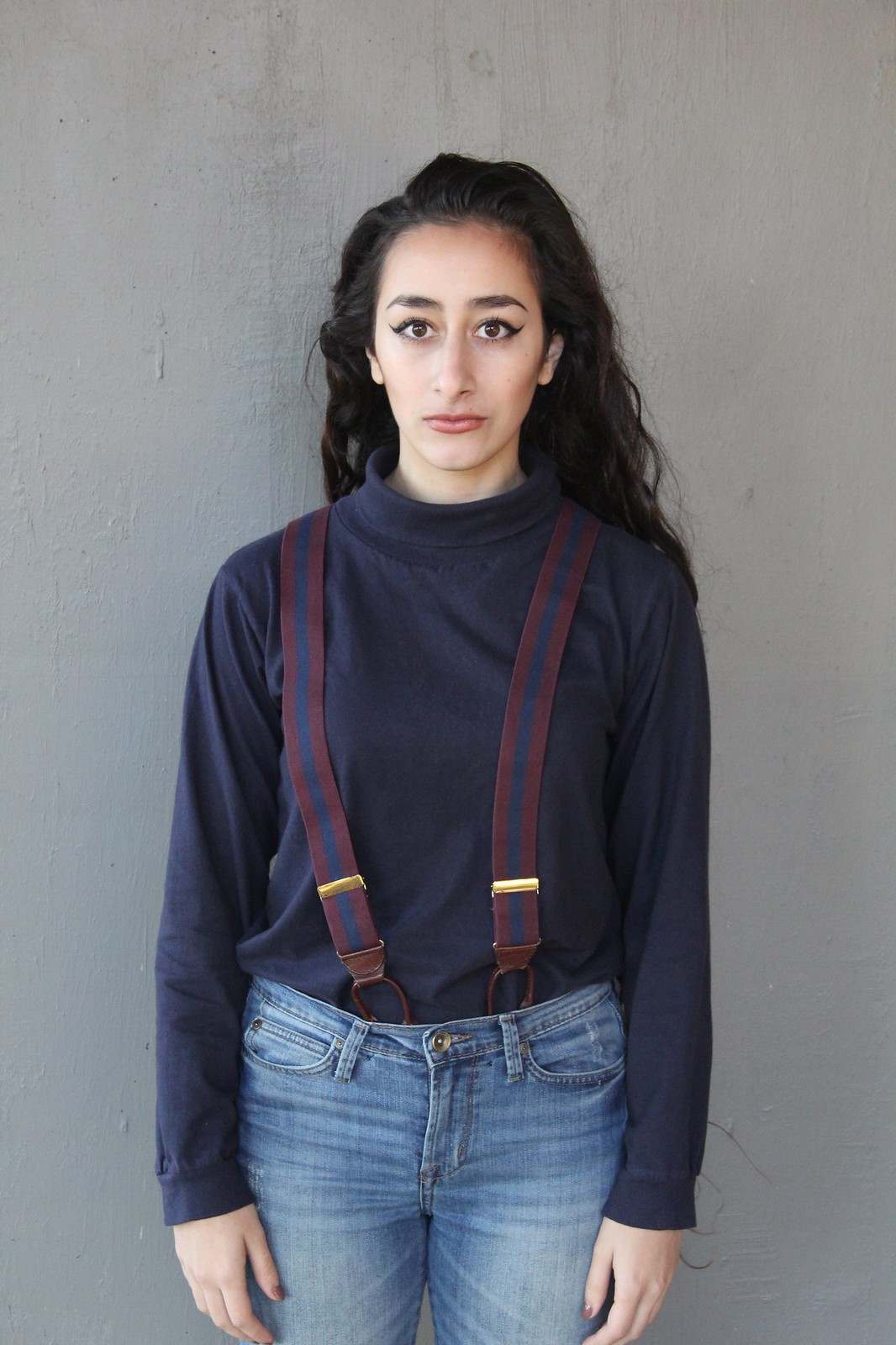This photograph features a young woman, estimated to be between 18 and 25 years old, standing solemnly in front of a textured gray stucco wall. The image is captured from mid-thigh up, showing her full attire. She is dressed in blue jeans and a long-sleeved black turtleneck shirt, complemented by a pair of suspenders that are striped with maroon and dark blue and have gold or copper clips. Her long, wavy, almost black hair is neatly combed back and tucked behind her shoulders, framing a face adorned with bold makeup, including extended winged eyeliner, mascara, and lipstick. Her fingernails are also polished. With her arms at her sides and her gaze directed straight at the camera, she exhibits a serious, emotionless expression.